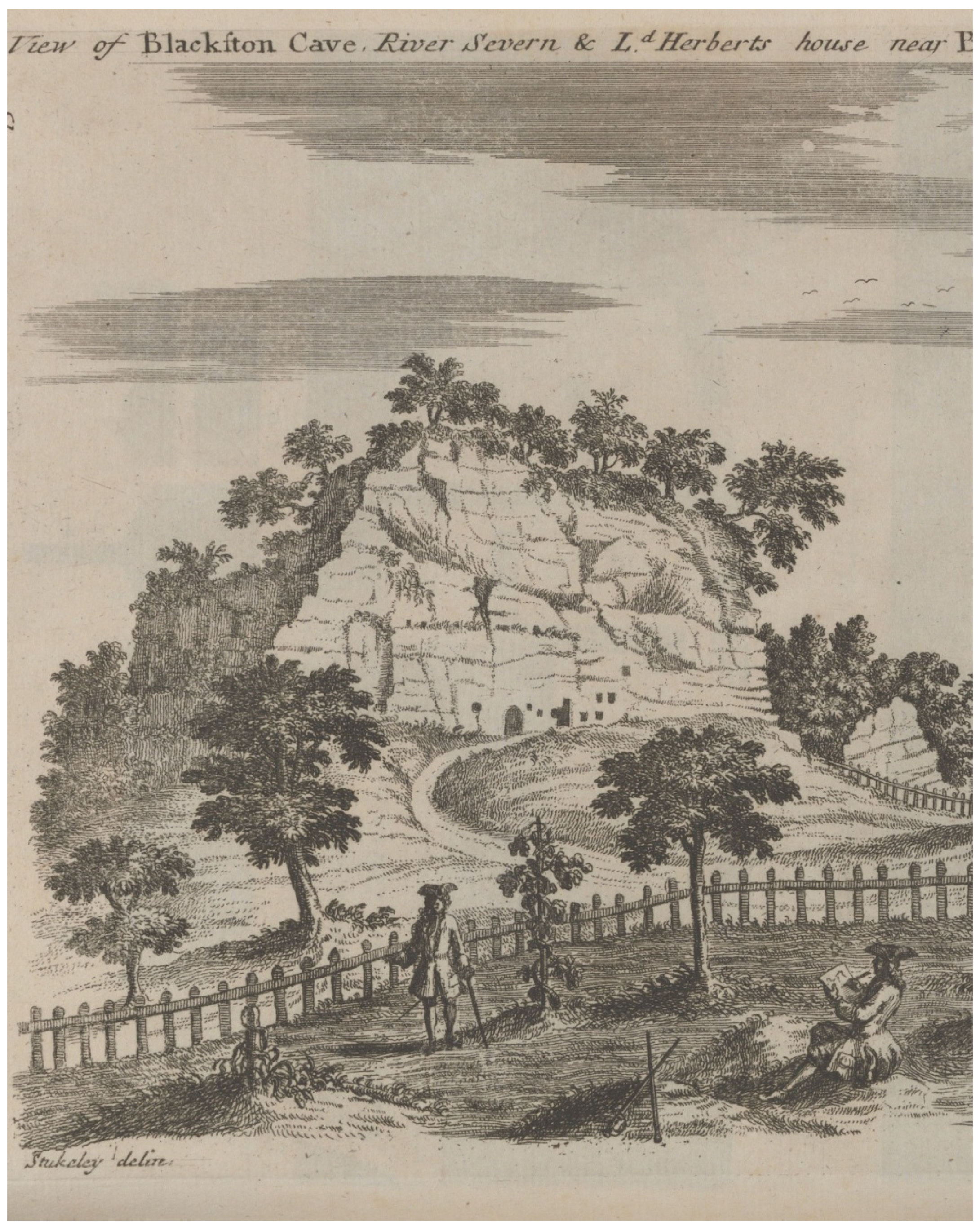This detailed black and white pencil sketch, rendered on light brown sketch paper or parchment, likely from the early 1700s, depicts a historical countryside scene. In the foreground, a wooden picket fence stretches horizontally, forming a boundary between the two main figures and the hilly terrain behind them. On the right, a seated woman in pre-colonial attire — a blouse, skirt, and British hat — is deeply engrossed in sketching with a pencil in her right hand and holding a drawing pad in her left hand. Adjacent to her, a man dressed in traditional British explorer clothing, including a vest and a British hat, stands with a cane in his left hand, appearing engaged in what might be observation or yard work.

The landscape extends beyond the fence, revealing a tall, rocky bluff or mountain with scattered trees and a small settlement structure carved into its base, complete with a door or an archway. Further detailing the background, the image hints at a serene natural environment with grasses, a pathway, and clouds dotting the sky. At the top of the image, partially visible text reads, "View of Blackton Cave, River Siren, and L Herbert House near." The drawing emphasizes the harmony between human activity and the natural scenery, capturing a moment in time with remarkable attention to detail.